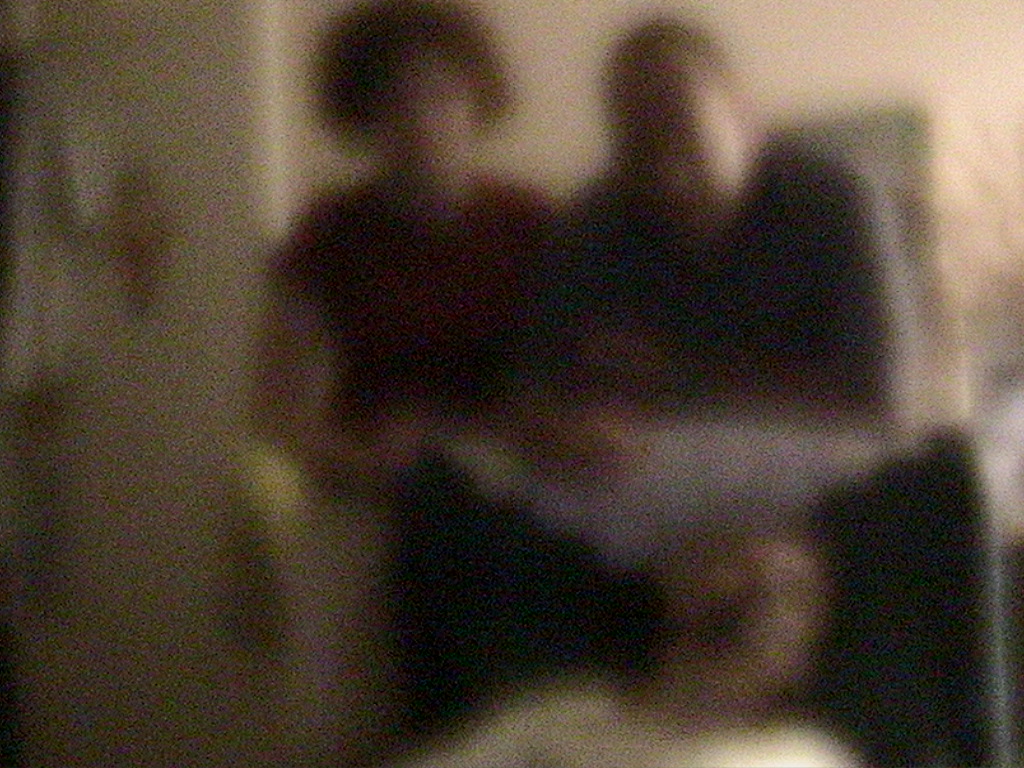In this slightly unfocused image, a serene scene unfolds against a light-colored, possibly beige wall. At the center, a person dressed in a white t-shirt is seen sleeping in a large, cushy chair adorned with a small white doily draped over its backrest. Behind the chair, two individuals stand watching the sleeping person. One is dressed in a long-sleeved shirt, while the other wears a short-sleeved, red-hued shirt. They both lean gently on the chair, creating a protective and watchful ambiance. In the background, a doorway is visible, adding depth to the setting. Adorning the wall is an intriguing gold-and-white decorative piece, quietly enhancing the calm and intimate atmosphere of the scene.